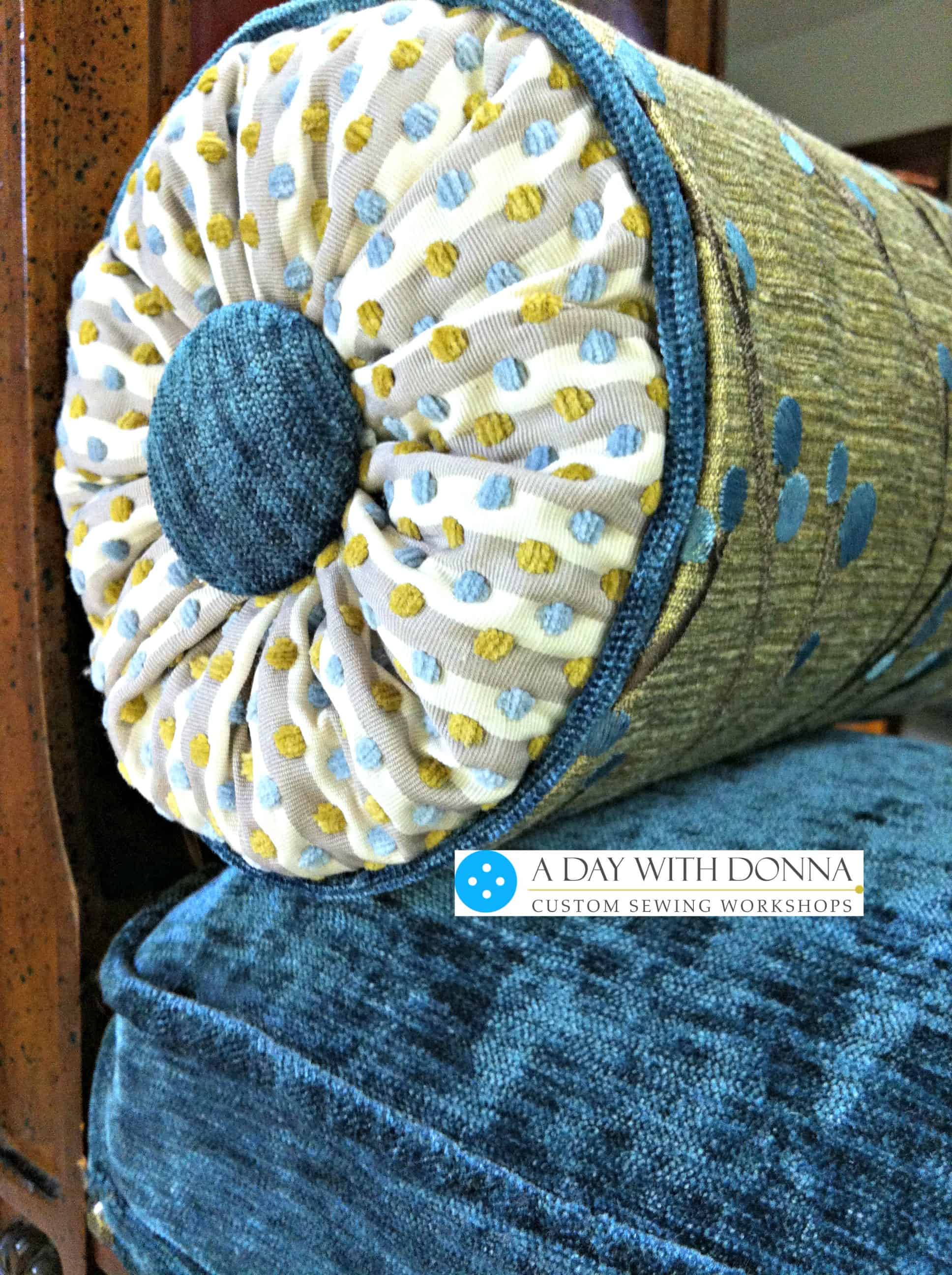In the image, two distinct throw pillows are placed against a dark brown wooden headboard with tiny black dots. The lower pillow is a velvety dark blue cushion featuring light blue squares and ridges around its edges, lending it a plush and soft texture. Positioned above it is a cylindrical cushion with an intricate design: it has a rough yellowish exterior with thin horizontal blue lines and spots, transitioning into a white section adorned with blue and yellow dots that crinkle towards the center. The center of this cushion showcases a dark blue circle that matches the pillow beneath. The setting appears to be indoors, and across the middle of the image, there’s a sign in a white rectangle with a blue button, reading "A Day with Donna Custom Sewing Workshops."